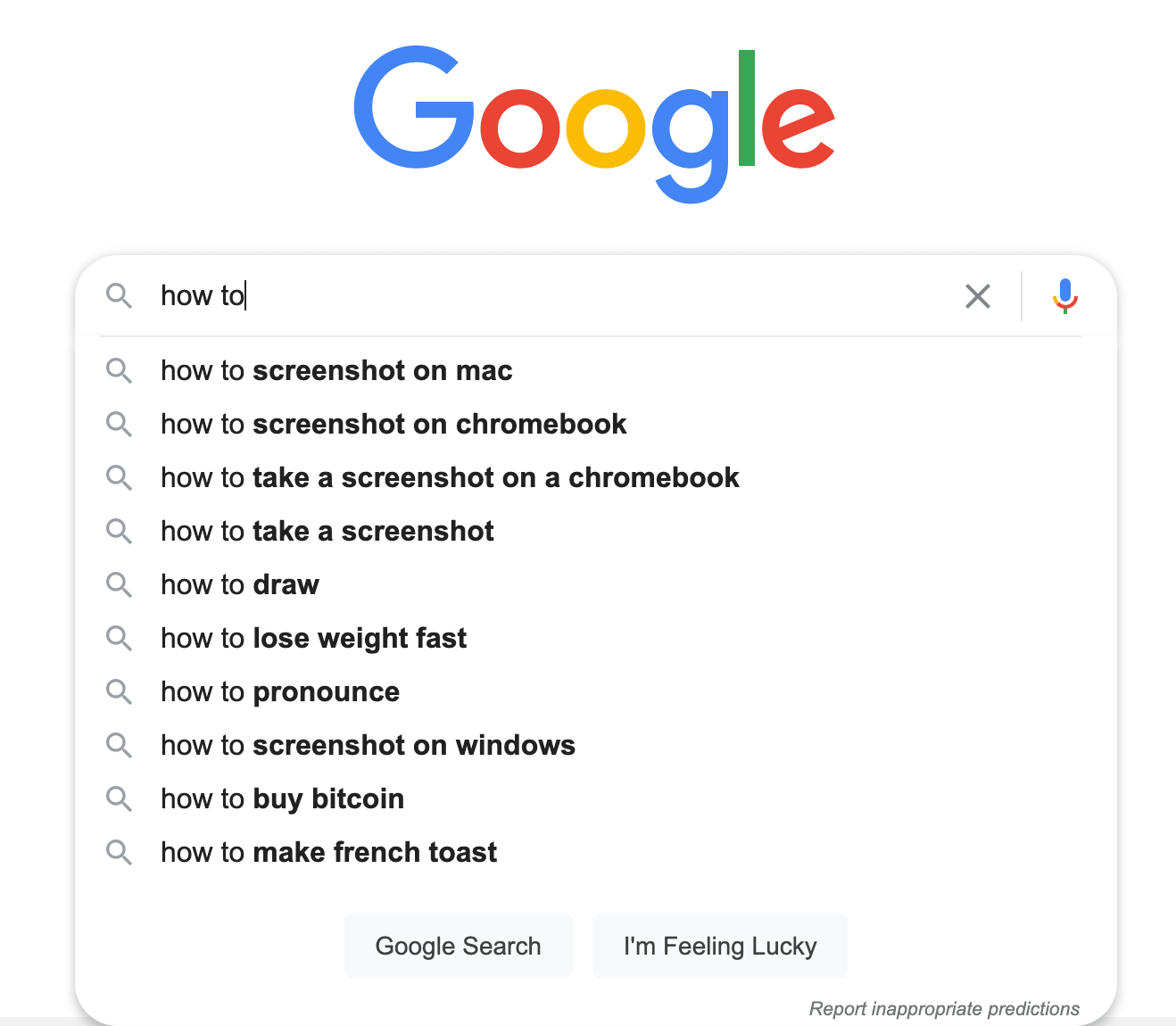The image is a screenshot of a search engine page titled "Gokli." The "Gokli" logo at the top displays in four colors: the first 'G' is blue, the first 'O' is red, the second 'O' is yellow, the second 'G' is blue, the 'L' is green, and the 'E' is red. Directly below the logo is a search box with a 'how to' query entered, and a series of auto-suggestions appearing beneath it.

To the right of the search box is an 'X' icon to clear the search, followed by a microphone icon in Gokli's signature colors, allowing users to record voice searches. On the left side of the search box is a search button depicted as a magnifying glass.

The auto-suggestions listed under the search box include:
1. How to screenshot on Mac
2. How to screenshot
3. How to screenshot on Chromebook
4. How to take a screenshot on Chromebook
5. How to take a screenshot
6. How to draw
7. How to lose weight fast
8. How to pronounce
9. How to screenshot on Windows
10. How to buy Bitcoin
11. How to make French toast.

Below the search suggestions are two grey buttons with white text. The button on the left reads "Gokli Search," while the button on the right reads "I'm Feeling Lucky."

In the bottom right corner of the image, there is italic grey text that reads "Report inappropriate predictions," offering users the option to report any unsuitable suggestions provided by Gokli.